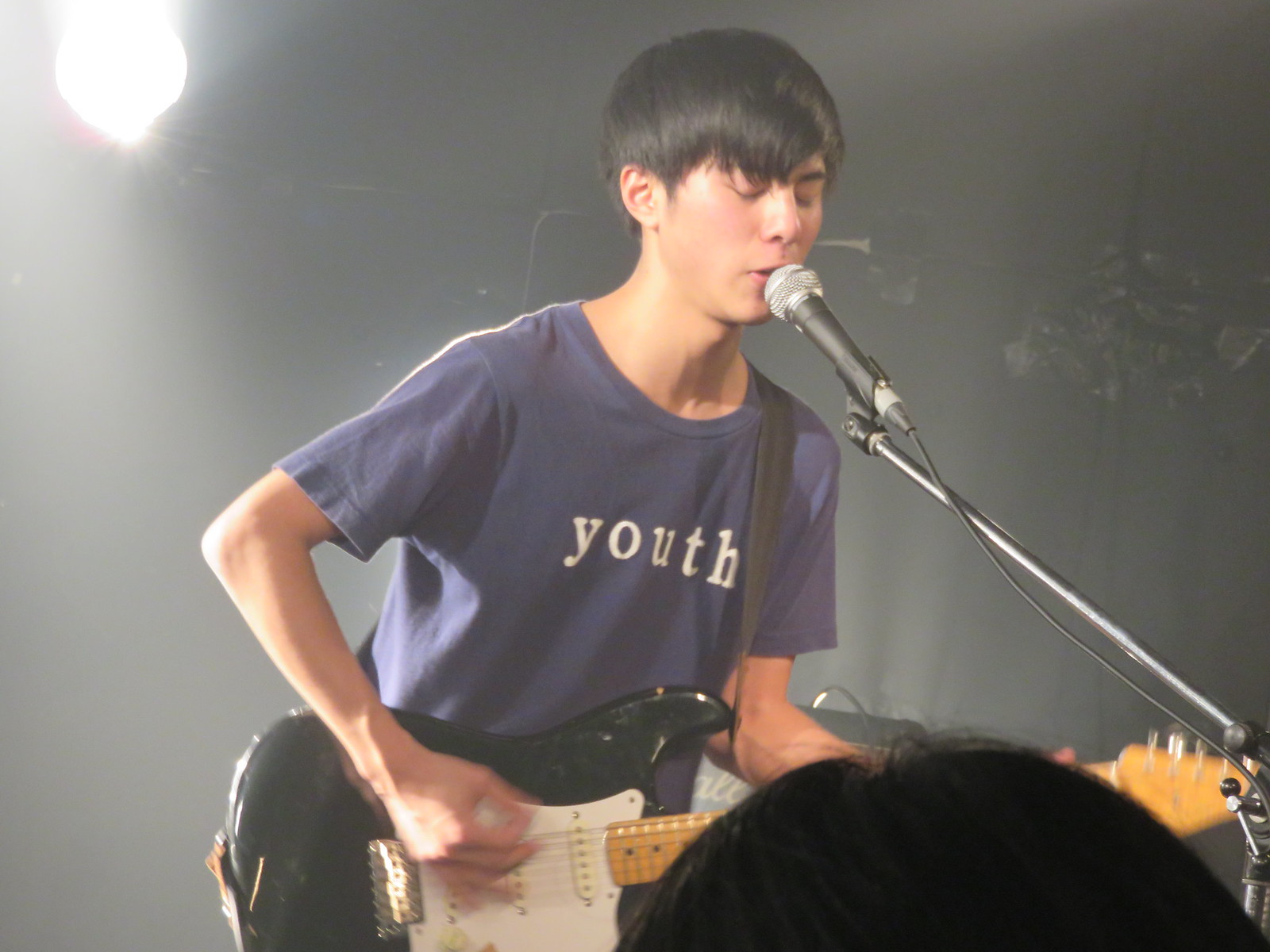In this color photograph, set in a dimly lit indoor environment, a young Asian man, around 15 years old, stands at the center as the primary focus. He has jet black hair styled in a bowl cut with bangs slightly covering his face and his eyes closed. He is captured mid-performance, singing into a black and silver microphone mounted on a stand while playing a black electric Fender or Squier Stratocaster guitar with a white pickguard and pickups, and a maple neck. His dark blue t-shirt bears the word "youth" in bold, white lowercase letters across his chest. A bright spotlight illuminates the top left corner, casting a sharp light in the otherwise hazy gray and black background. The back of a woman's head with black hair is partially visible in the bottom right corner of the image. The overall composition depicts the authentic atmosphere of a music concert, highlighting the intensity and emotion of the young musician's performance.